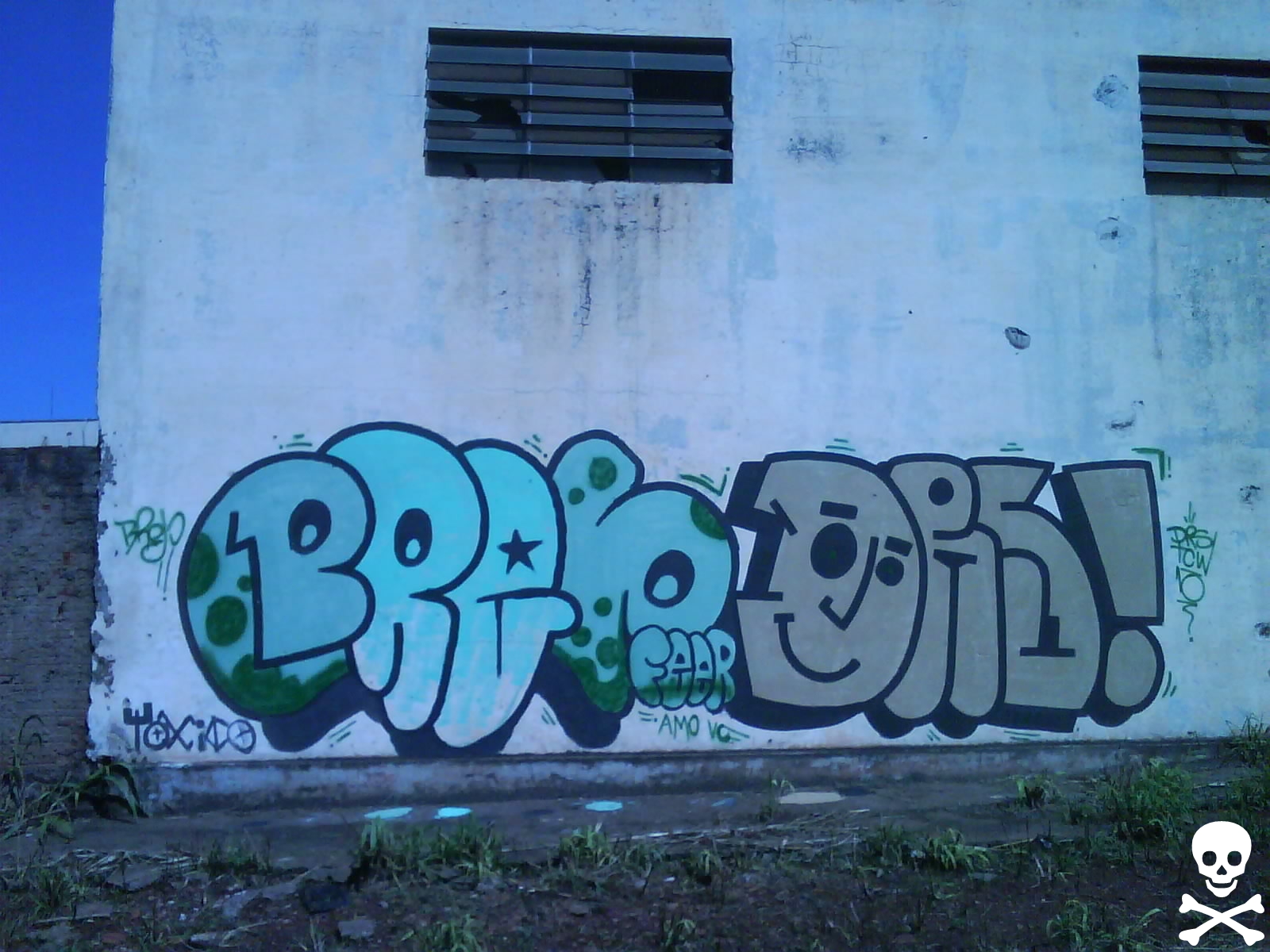The color photograph, taken outdoors in a landscape orientation, depicts the side of an old, white-rendered building, showing significant signs of age and neglect with prominent yellow stains, blue marks, and various forms of damage. The building features two upper windows with dark, tinted and partially broken glass, one centrally located and the other cut off on the far right. 

The lower portion of the building showcases an array of graffiti in stylized block letters with black outlines. The hues transition from shades of blue and turquoise to green and grey, ultimately forming an indecipherable message, although parts of it clearly spell "FEAR" in blue and "AMO" in smaller black font. There's an exclamation point at the end marked in a reddish tone, which adds a dramatic flair to the graffiti.

A pristine blue sky can be seen on the far left of the photograph, enhancing the outdoor setting, while the base of the building and ground cover a mix of dirt and sparse green weeds. A comical skull and crossbones motif, superimposed in white, resides in the bottom right corner of the image, adding an element of whimsy to the otherwise gritty scene.